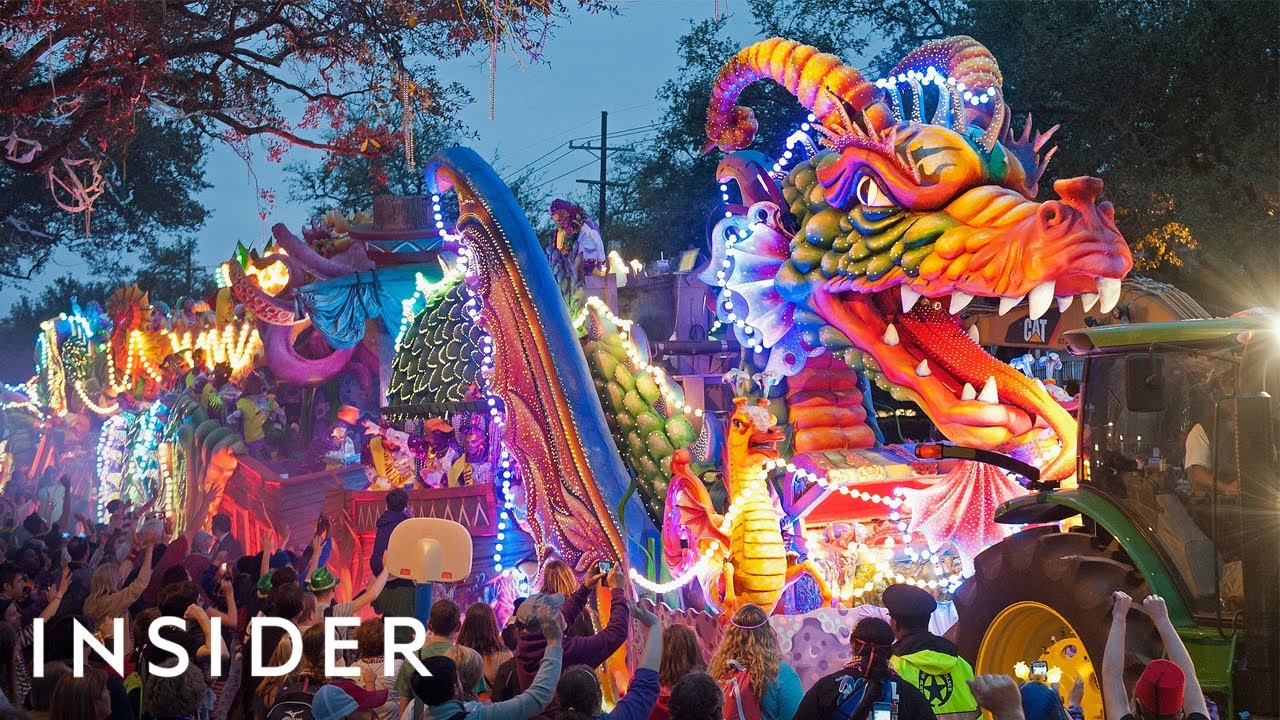Against the backdrop of an evening sky transitioning to deep blue, a vibrant carnival parade unfolds in this captivating image. Dominating the scene is an expansive float in the shape of a dragon, its colorful body—adorned in hues of yellow, green, blue, and purple—stretching from the right of the picture to the left and illuminating the night with numerous lamps and lights. A bustling crowd lines the street, their backs facing the camera as they capture the spectacle with their cell phones. Among them, a policeman in bright yellow rain gear, identifiable by his cap, stands out. The float’s dragon head is a striking feature with its enormous white teeth, open jaws, red nose, and prominent horns, situated near a John Deere tractor that seems to be pulling it. Additional carnival rides and vibrant decorations are visible in the background, contributing to the lively atmosphere. The bottom left corner of the image contains small white text reading "INSIDER," hinting at the possibility of a magazine coverage.